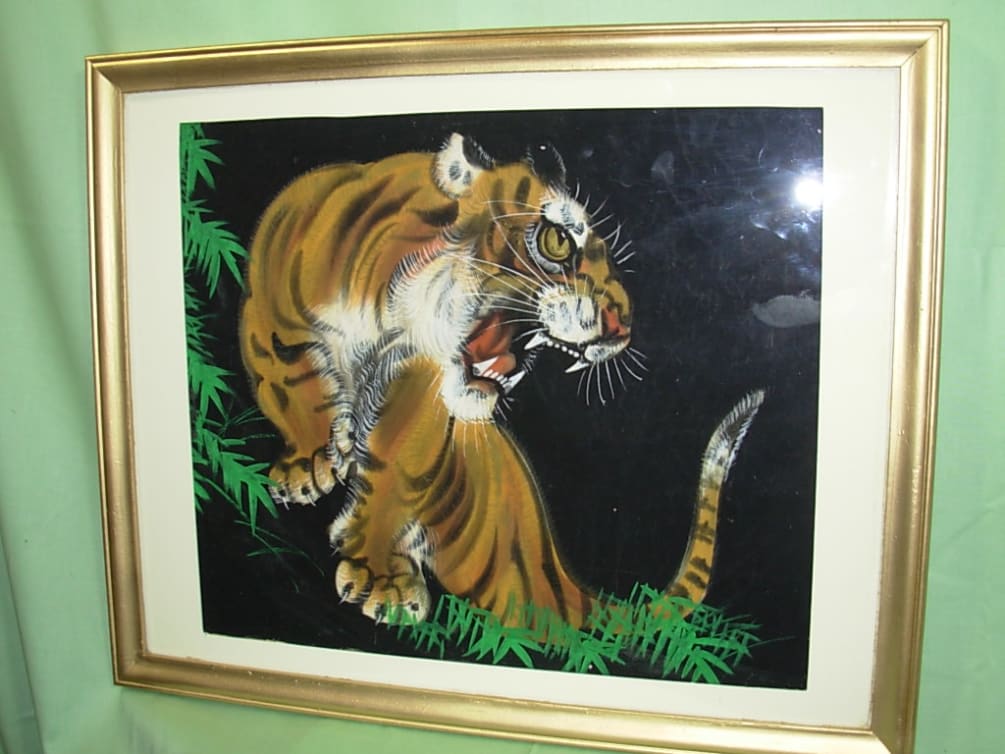This image captures a striking painting of an orange Siberian tiger, framed and displayed with notable intensity. The tiger, painted on a black background, is showcased within a golden-colored frame that features a white mat. Set against a light green wall, the artwork's presentation is somewhat marred by the reflection of a camera lens flash in the top right corner and visible fingerprints on the protective glass. The tiger itself is depicted in a dynamic pose, its head turned to the right with its mouth wide open in a fierce growl, showcasing sharp, prominent fangs. The creature's yellowish eyes are intense and focused, with its ears pointed outwards. Its front paws, robust and massive, rest on a dark branch, surrounded by green foliage resembling palm leaves. This scene evokes a sense of tension, as though the tiger is either defending itself or poised to pounce, exuding a palpable aura of raw power and alertness.